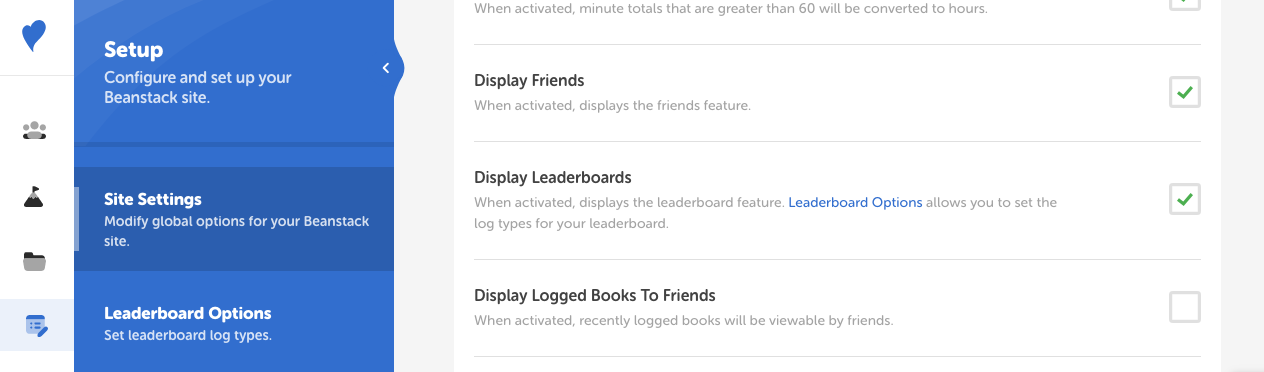This screenshot displays a website configuration interface specifically structured for setting up and customizing a Beanstack site. The image is wide and horizontally oriented, with an approximate aspect ratio of 20:80. 

On the left side, a vertical sidebar features a series of icons: a small, blue wavy heart, a group of people, a mountain with a triangle on top, some folders, and a calendar with a pen. Each icon is indicative of different sections or functionalities of the site.

Adjacent to the sidebar, a prominent blue rectangular section contains white text with bold titles, providing various setup options for the Beanstack site. The options listed include:
- **Setup**: Configure and set up your Beanstack site.
- **Site Settings**: Modify global options for your Beanstack site.
- **Leaderboard Options**: Set leaderboard log types.

To the right of this section is a gray background area featuring further configuration descriptions in white text. These settings include:
- **When activated, minute totals that are greater than 60 will be converted to hours**.
- **Display Friends**: When activated, displays the friends feature.
- **Display Leaderboards**: When activated, displays the leaderboard feature. A hyperlink labeled "Leaderboard Options" offers additional configuration for log types.
- **Display Log Books to Friends**: When activated, recently logged books will be viewable by friends.

This detailed layout ensures that users can effectively manage and personalize their Beanstack site with a variety of options to enhance user experience and engagement.